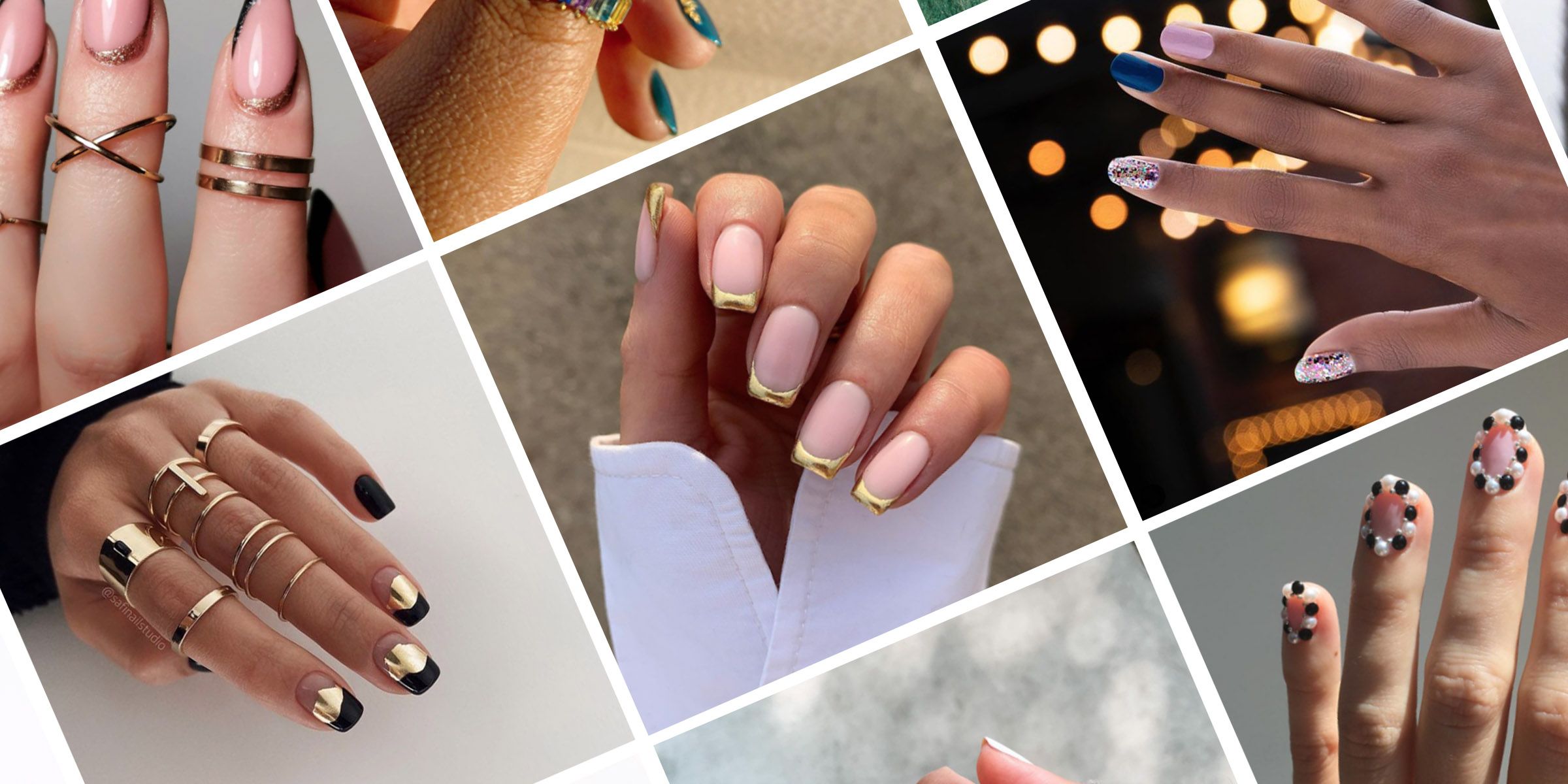The photograph is a detailed collage exhibiting close-ups of meticulously manicured women's fingernails, arranged in seven diamond-shaped images. Each panel highlights different intricate nail art designs and the adorned fingers of Caucasian women. Centered in the collage, a woman showcases a French manicure with lustrous gold tips, complemented by a white-collared shirt cuff. The bottom left panel features a hand adorned with numerous gold rings and nails painted in a gradient of clear to bright gold, finishing with black tips, and a solid black pinky nail. Other panels display various artistic designs, such as nails painted with glitter, navy blue, and light pink; one even incorporates tiny beads as embellishments. This collage, likely an advertisement for a nail salon, captures the range of sophisticated techniques and styles available.